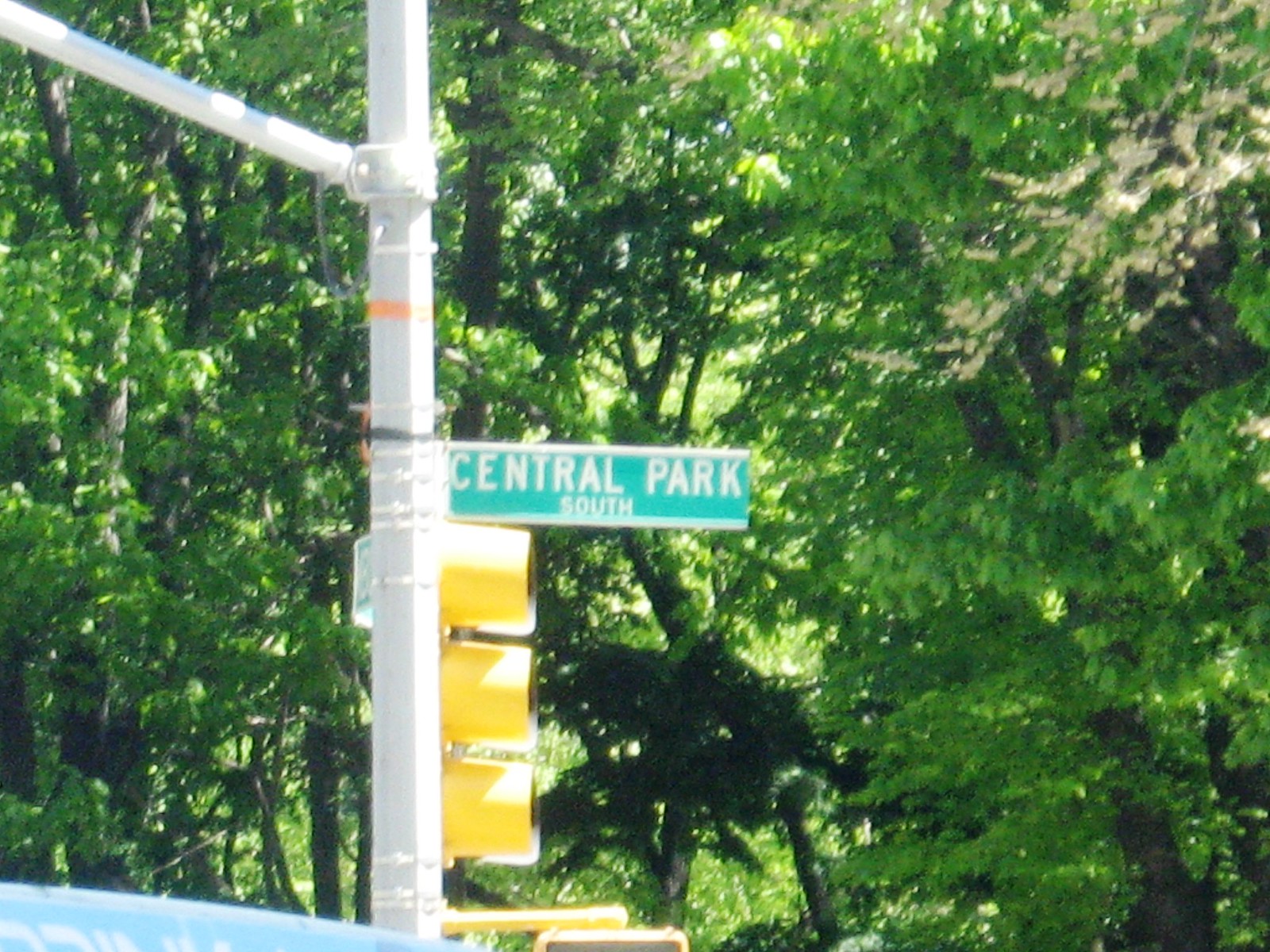The photograph, taken outside on a bright sunny day, showcases a bustling intersection with a prominent gray metal pole dominating the scene. This pole, located off-center to the left, features several straps supporting various signs. Prominently displayed near the top of the pole is a green street marker with bold, white letters reading "Central Park" and smaller text below it stating "South." Below this, a three-tiered stoplight array presents itself from a side view, revealing its yellow lights, while just beneath, a pedestrian signal with a yellow frame and black screen is visible. Extending horizontally near the top of the pole is a silver bar. The bottom left corner of the image hints at a blue piece of metal, likely part of a car, adding a subtle urban touch. The background is lush with greenery, showcasing numerous trees with leaves in various shades of green due to the sun's reflection. Among these, a tree boasting white blooms, possibly hawthorn, stands out in the upper right corner, with dark trunks providing a striking contrast to the vibrant foliage. A sliver of blue sky adds to the bright and lively atmosphere of the park scene.